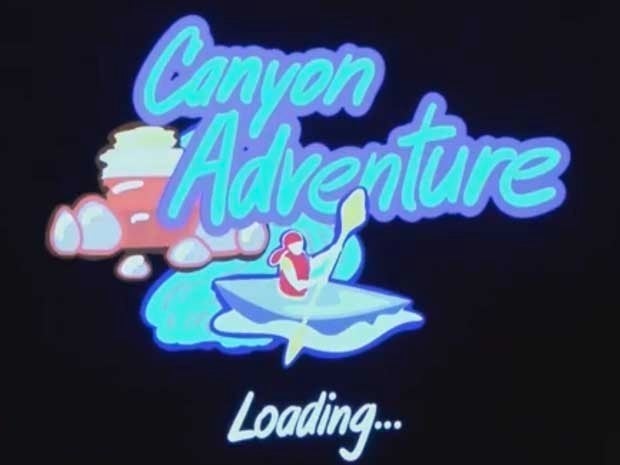The image features a bold, dynamic graphic set against a solid black background. At the top center, light blue text outlined in a darker blue reads "Canyon Adventure." Below this title, a captivating illustration depicts a person in a canoe, energetically paddling with yellow oars through blue waves. The paddler is wearing a distinctive red vest with yellow shoulders and a matching red cap. To the left side of the canoe, an array of gray rocks adds rugged texture to the scene. At the bottom center of the image, the phrase "Loading..." appears in white text, indicating a transitional or preparatory stage. The design strikes a balance between adventure and anticipation, inviting viewers into the vivid world of a thrilling canyon escapade.